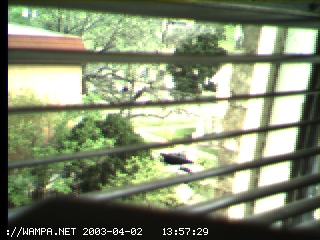This image is an unfocused, small color photo, likely captured from a security camera, dated April 2, 2003, at 1:57:29 PM. The photo displays a view from inside a house looking out through horizontally slatted Venetian blinds. The window reveals an outdoor scene: the bright sunlight highlights a back or front yard with various elements. To the right, a little bit of a white window sill is visible, and to the left, part of a brick wall. Dominant in the scene are tree trunks, shrubs, and large green trees, suggesting a sunny day. In the bottom section of the image, there's a glimpse of grass and possibly a driveway with the faint outline of a black truck. Above, near the center-left, is a yellow building with a red roof, partially obscured by a thick green tree branch. Further details include the side of a structure, potentially a garage or shed, amidst more trees and greenery, with a lightly visible road running across in front of the yellow house.